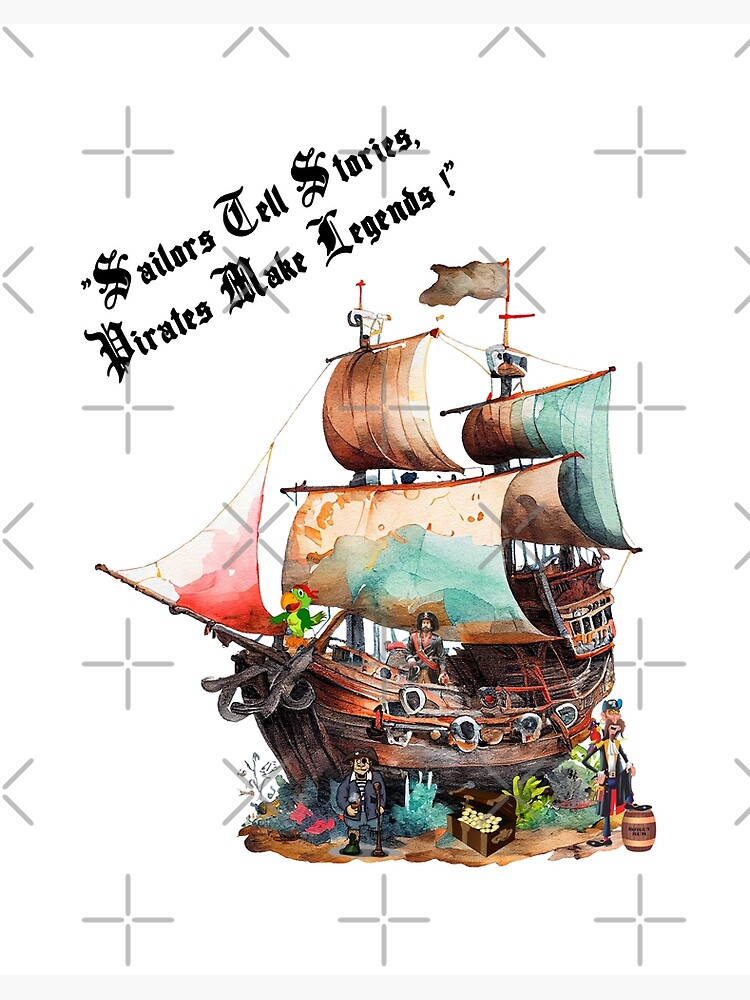The artwork features a cartoonish depiction of a pirate scene set against a plain white background adorned with light gray pluses and Xs that resemble a watermark. In the upper left-hand corner, a black-inked diagonal quote proclaims, "Sailors tell stories. Pirates make legends." 

At the heart of the image stands a grand pirate ship with a brown body. It boasts several sails of various colors including brown, light green, and one decorated with a map. Prominently in the middle of the ship is a pirate donning a hat. Toward the front of the vessel, a vibrant green parrot with a red wrap perches beside a red sail, while its dark green wings and orange beak add more character. 

On the ground in front of the ship, a gathering of pirates surrounds piles of treasures, completing the lively pirate tableau.